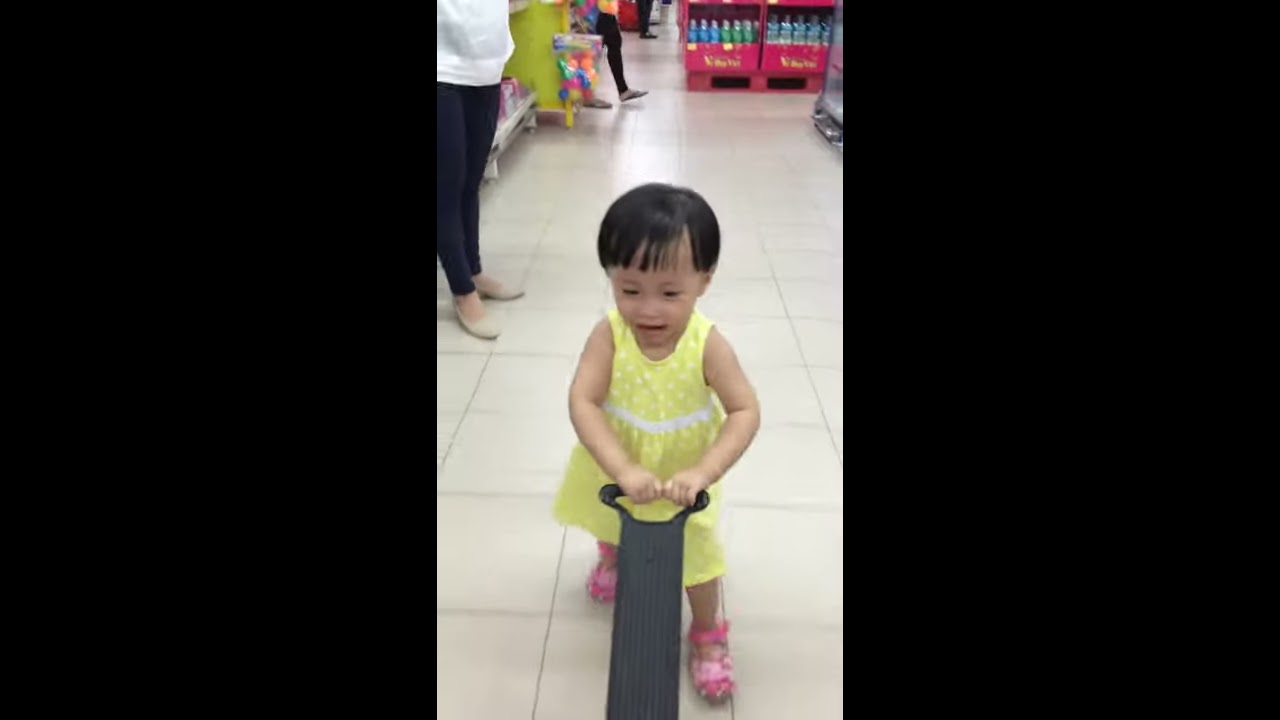In the center of the grocery store interior, a young Asian toddler with short black hair is captured wearing a charming yellow dress adorned with white polka dots and a white belt. Pink sandals grace her tiny feet as she pushes a black child cart toy with both hands. The grocery store floor is clean, consisting of large gray and tan tiles. To the left of the child stands an adult woman, likely her guardian, dressed in tight black pants, a white shirt, and tan flats. The aisle to the left features shelves stocked with various products and notably has plastic toys hanging in a bag from the side of the shelf. Further down the aisle, a red display showcases an assortment of blue and green bottles. In the background, additional shoppers can be seen walking down the aisle, contributing to the busy ambiance of the store. The focal point, however, remains the delightful scene of the young girl joyfully navigating her cart through the store.